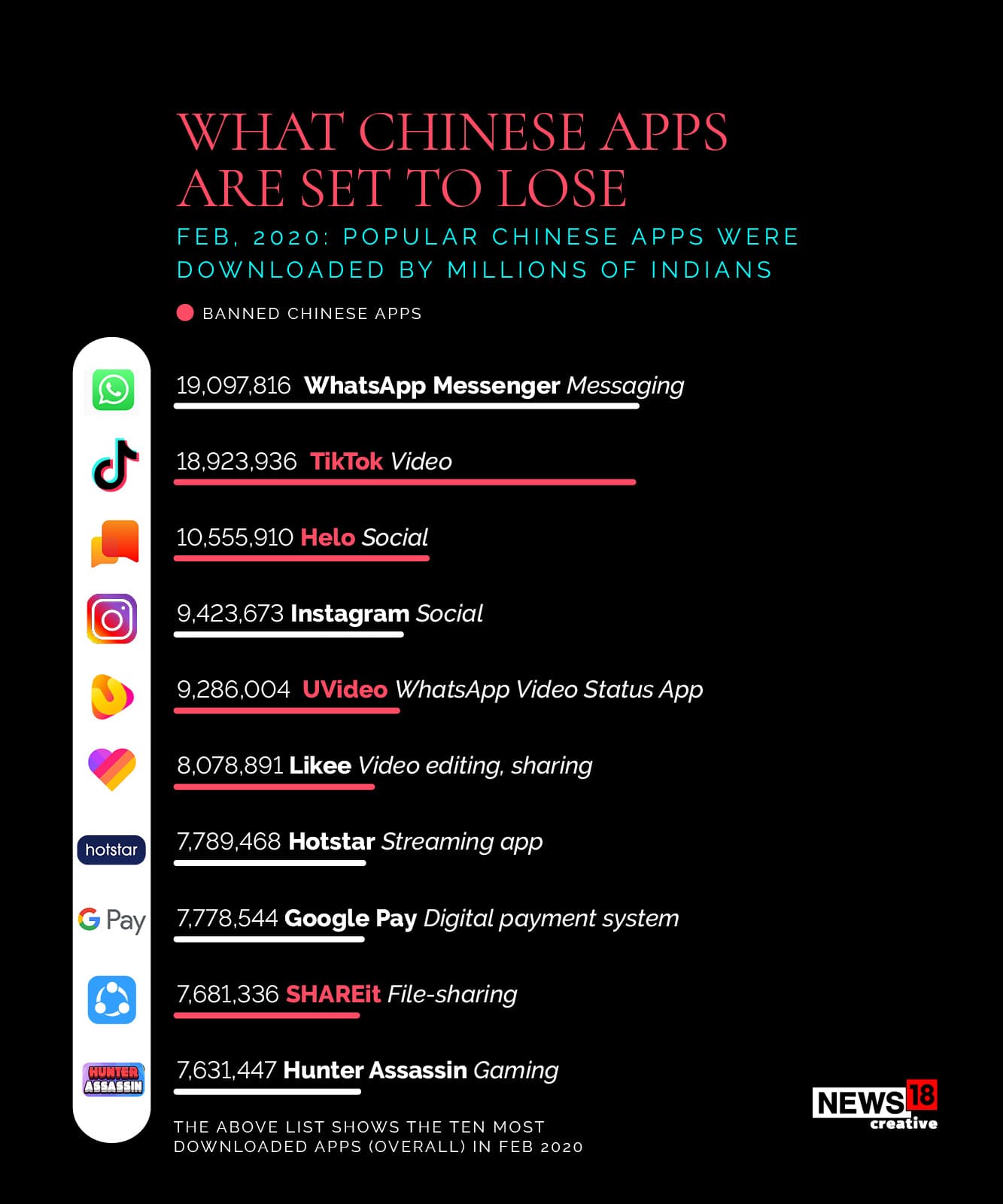The image features a solid black background with various texts and icons overlaid. At the top, in bold red text, it reads: "What Chinese Apps Are Set to Lose?" Directly beneath this, in vibrant turquoise lettering, the caption states: "February 2020 popular Chinese apps were downloaded by millions of Indians."

In the lower portion of the image, there is a large, solid red circle containing the phrase "Banned Chinese Apps" in white text. Within and around this circle, a list emerges, highlighting several notable apps: WhatsApp, TikTok, Helo, Instagram, YouVideo, Likee, Hotstar, along with Gpay, Shareit, and a mention of "Hunter Sessom Gaming, News18 Creative."

The image is further augmented with icons representing WhatsApp, TikTok, Helo, and Instagram, visually reinforcing the apps mentioned. The caption at the bottom elucidates that the list identifies the ten most downloaded apps overall in February 2020.